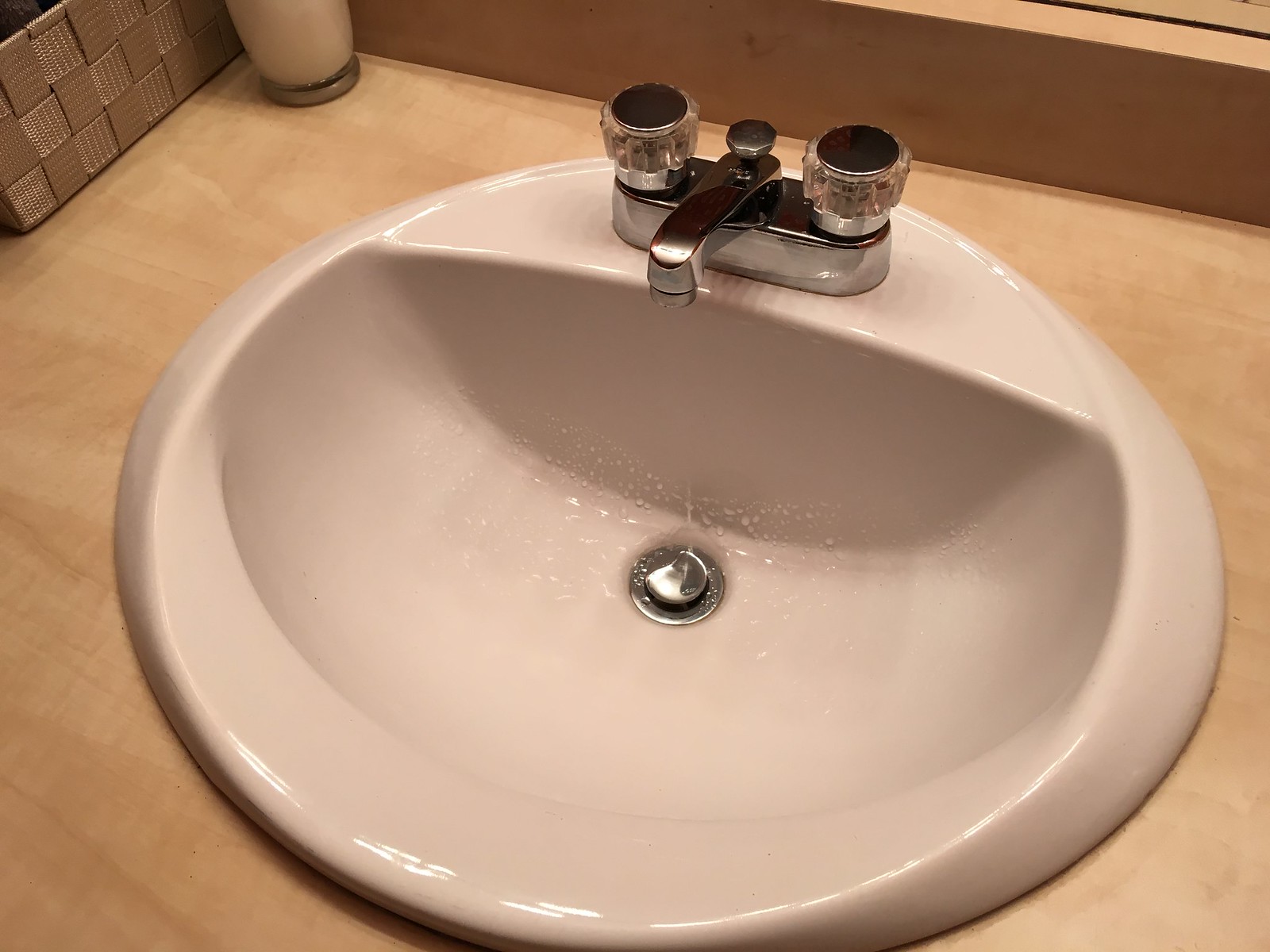This is a detailed photograph of a bathroom sink featuring an off-white, slightly dirty-white, oval-shaped porcelain basin with a thick lip. The sink is equipped with a hot and cold mixer tap that sits on a unified silver fixture with crystal-like twisting handles. The faucet in the center emits a slow, thin stream of water, and droplets have splashed at the base of the sink. The basin is set into a counter that appears to be a light brown wood laminate, mimicking the look of a grainy wood surface. 

In the top left corner, a fabric basket, possibly gold in color, is visible, along with what might be a brown jug on a silver stand and a glass container that could hold a candle. The top right corner of the image features the edge of a wooden frame and a hint of a mirror. The ambient light in the photograph is warm and subdued, casting a soft glow across the scene. The overall atmosphere suggests a mix of old-fashioned design elements and practical bathroom storage.